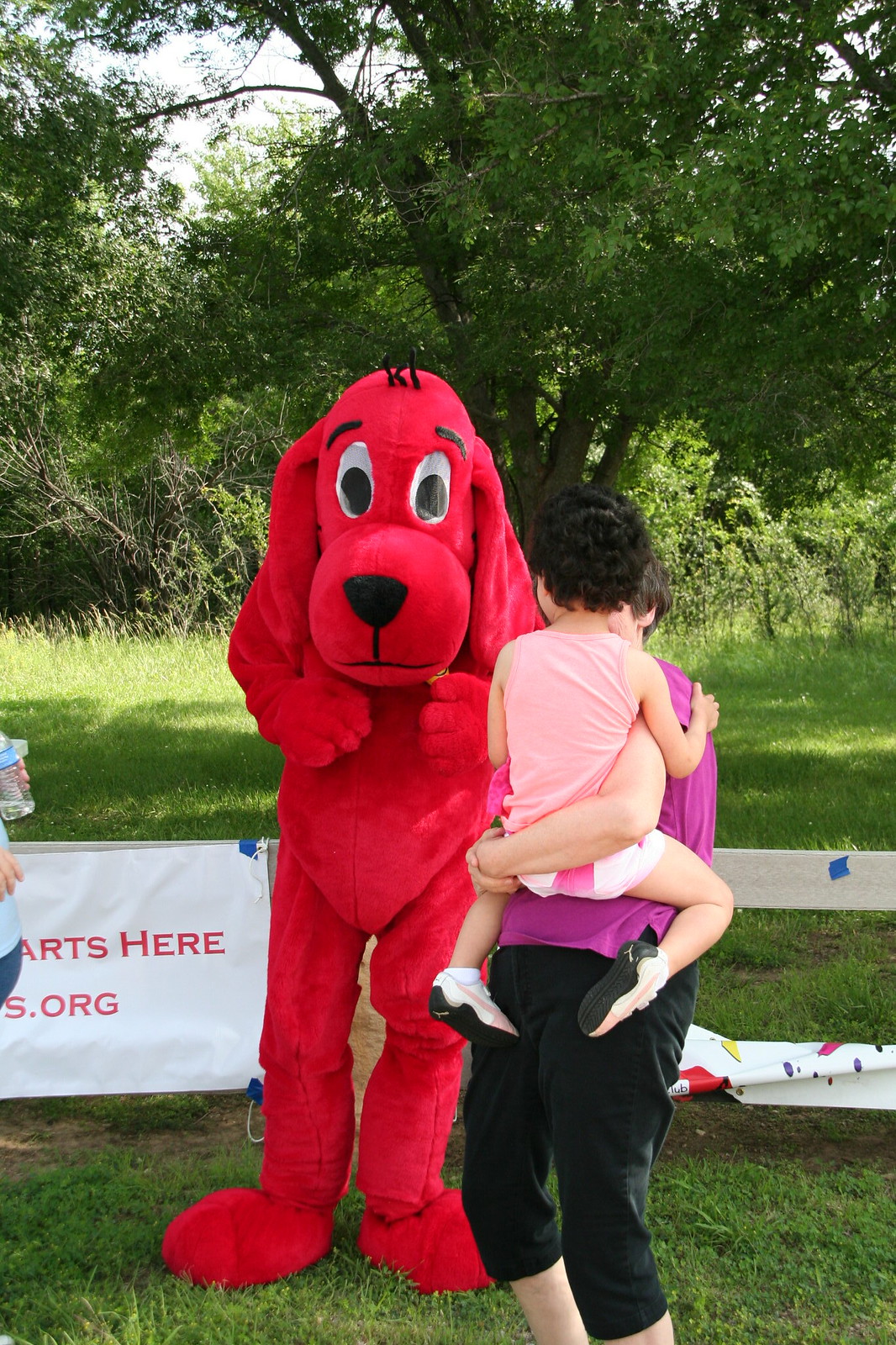This outdoor daytime photograph, taken in a park filled with green grass, tall trees, and a vibrant blue sky, captures a lively scene featuring a person dressed as Clifford the Big Red Dog. The bright reddish-orange dog suit boasts a serious but friendly-faced hood with white eyes and a black nose. Behind Clifford, a banner attached to a fence reads "ARTS here" and "S. dot org," indicating an open display or event, possibly a charity function.

In the foreground, a woman with dark curly hair dressed in black slacks and a pink top holds a large toddler facing away from the camera, looking towards Clifford. The toddler, also with dark curly hair, is dressed in a pink tank top, white shorts, and little sneakers. To the left side of the image, another individual partly appears, wearing a blue shirt and holding a clear water bottle. The scene is framed by well-mowed grass and shaded by a lush tree, adding to the picturesque setting.